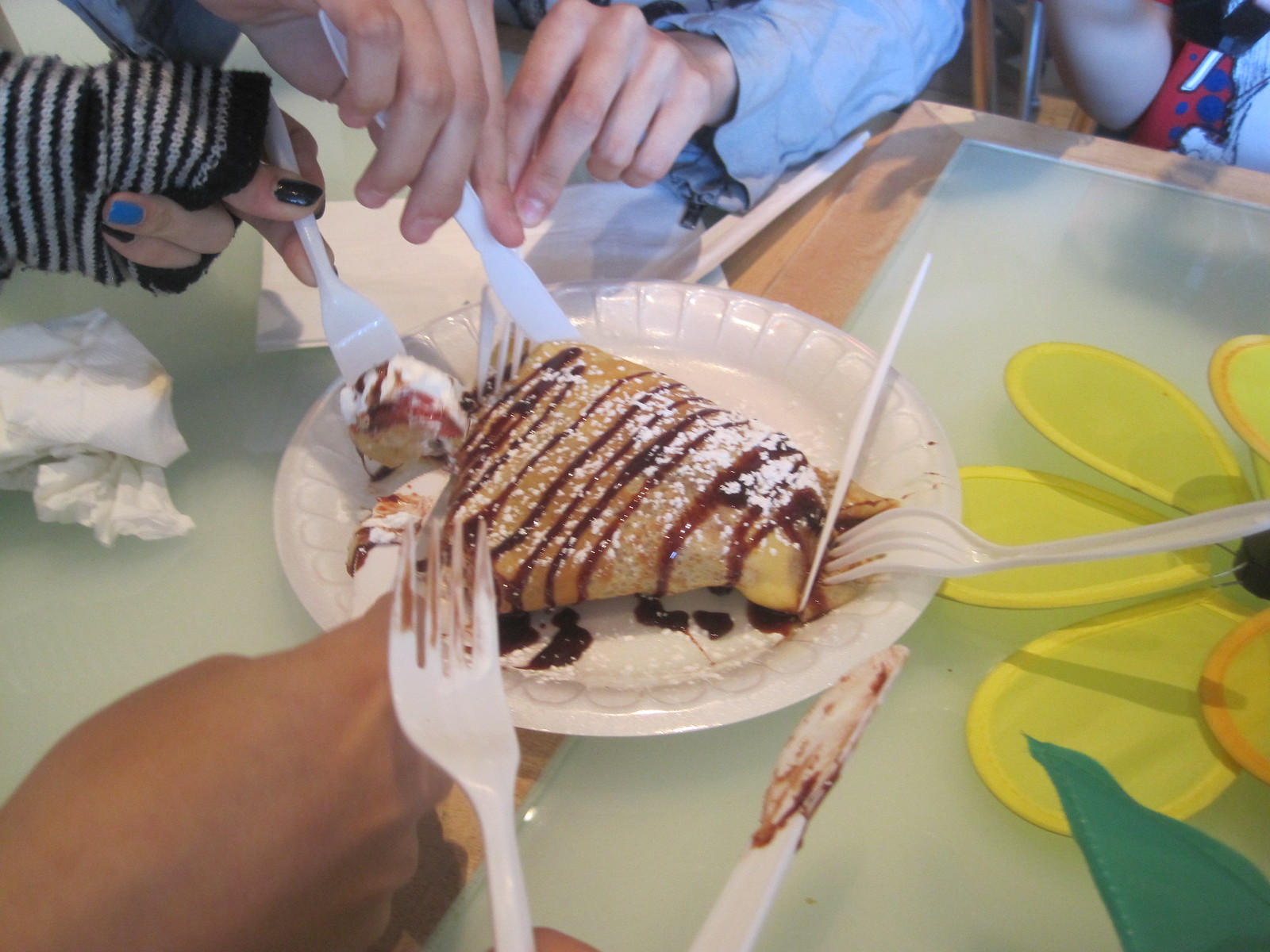In an indoor setting, a vibrant color photograph captures three people sharing an enormous, light brown crepe placed on a Styrofoam plate. The crepe, generously drizzled with raspberry syrup in neat lines and dusted with powdered sugar, has a golden-yellow hue suggesting a possible lemon or banana filling. The syrup has spilled slightly onto the plate itself, adding to the dessert's appeal. Surrounding the plate, various hands are actively cutting and serving portions of the crepe using knives and forks. One of the participants, a male in a wrinkled blue shirt, is prominently featured. To his side, a female with painted nails of black and blue, clad in a white and black striped sweater, reaches for a forkful. The dessert scene is further adorned with additional elements - scoops of white ice cream, a cutting board, napkins, a plastic sunflower, and an out-of-focus arm in the upper right corner. The atmosphere is buzzing with the immediate anticipation of enjoying the shared delight.